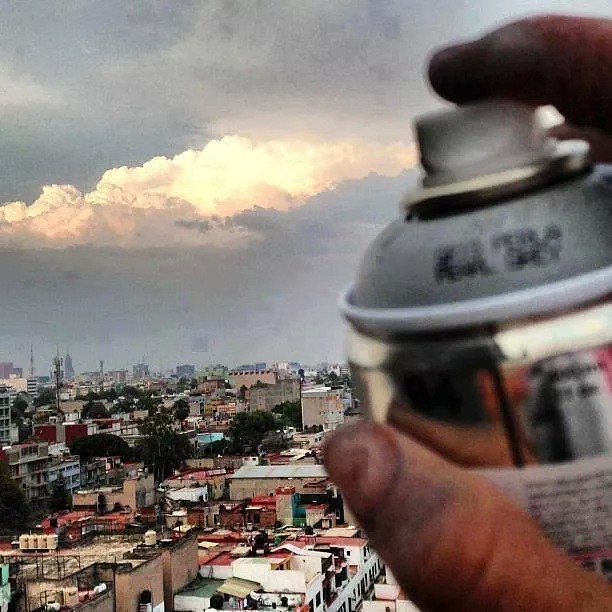Amidst a bustling urban landscape, an image captures the illusion of a man seemingly spray painting the sky. The perspective is from a high vantage point, overlooking a dense cityscape adorned with concrete buildings, meandering roads, and scattered trees. The sky above is a mix of vibrant hues, featuring fluffy white clouds tinged with gold and pink, interspersed with darker gray clouds that suggest recent or impending rain.

On the left side of the vertical image, a hand appears prominently in the foreground. It is slightly dirty and grasps a metallic spray paint can, with the person's thumb and finger curled around the container and their finger poised on the white nozzle. The can is angled to create the illusion that the person is spraying clouds into the sky, making it appear as though flames or clouds are emitting from the nozzle. This clever placement transforms an ordinary scene into a whimsical optical illusion, blurring the line between reality and fantasy.